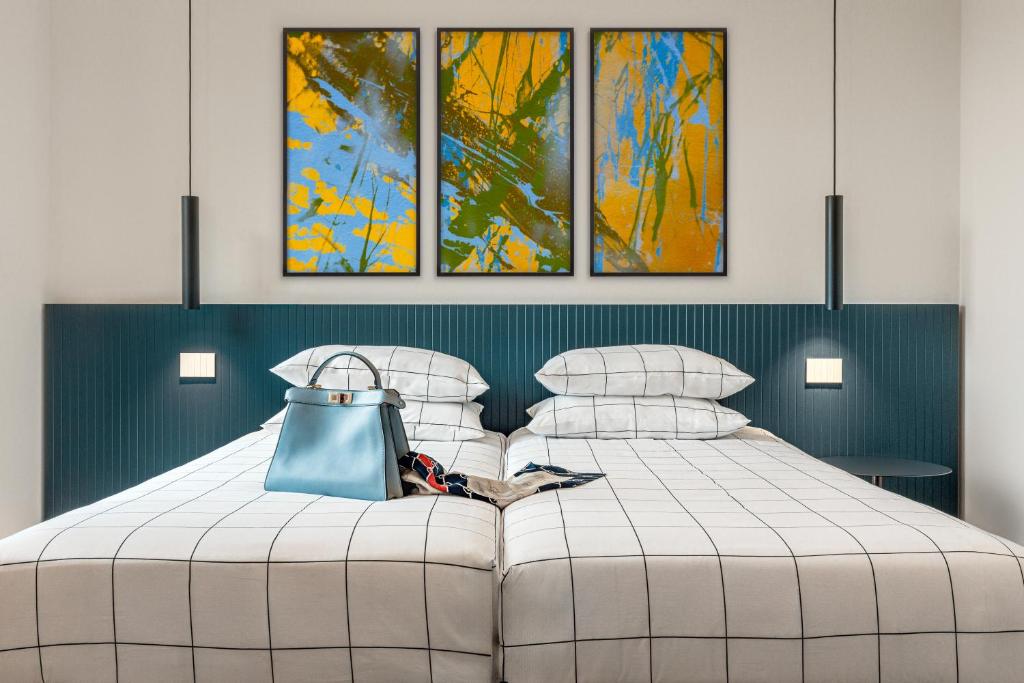This image depicts a hotel room featuring two twin beds pushed together, effectively creating a larger sleeping area. The room's walls are painted white with the lower half in blue. Above the headboard, which is a darker blue with recessed white vertical stripes, hang three abstract framed paintings in various shades of mustard yellow, green, brown, and light blue. These paintings, which look somewhat like Pollock's work but with thicker swathes of color, are in a triptych arrangement: the left painting has more light blue, the middle more green, and the right more orange.

Each bed is covered in white sheets with a navy blue square pattern and has two pillows adorned with matching pillow covers. At the foot of the leftmost bed, there's a light blue woman’s purse with a short strap and a silver fixture at the top. Next to it lies a blue and brown scarf with sections of grey and red, draped between the beds.

Flanking the beds are pendant lights hanging from the ceiling. These lamps, one on each side, have associated red-lit rectangles located just above and slightly outside the ends of the mattresses, adding a modern touch to the understated yet vibrant decor of the room. A small bedside table is positioned to the right of the right bed, further accentuating the modest, functional design of this inviting hotel bedroom.